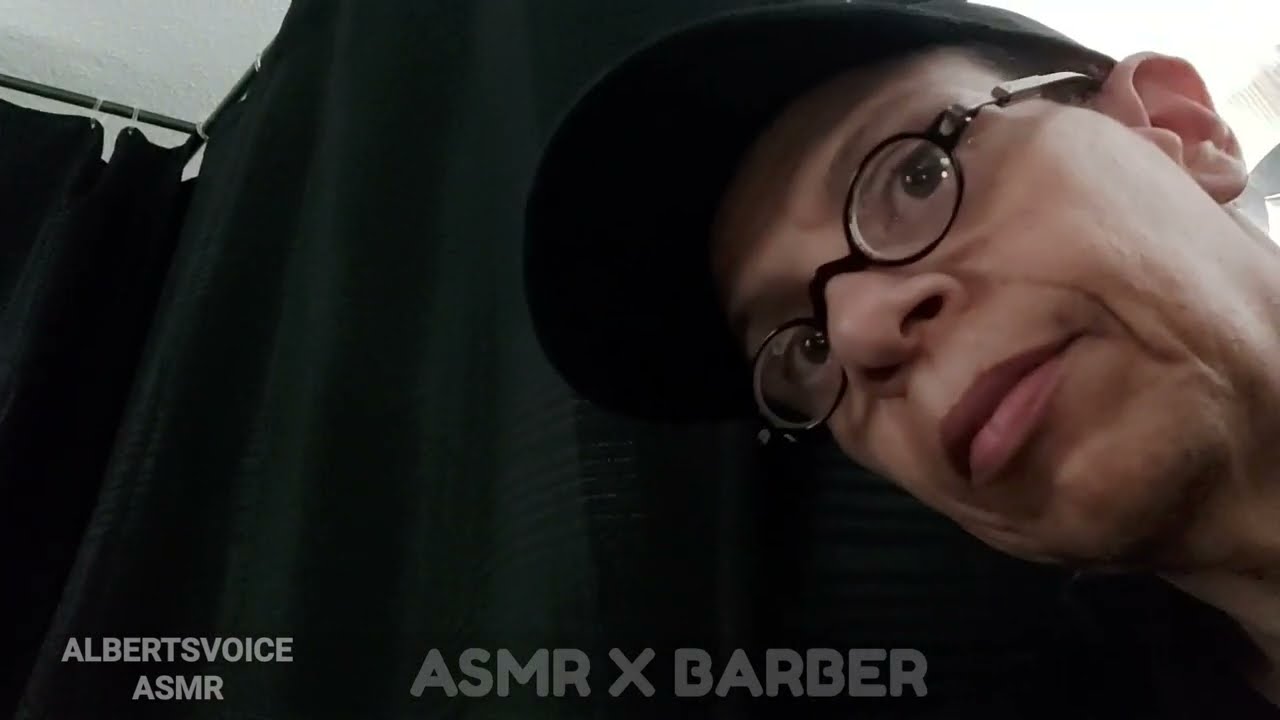This image features an older man, likely in his late 50s or early 60s, with Asian features. He is wearing a black baseball cap and black, oval-shaped glasses with thin frames. The man has a larger nose and prominent ears. He is looking directly at the camera without any particular expression. 

The background primarily consists of a dark green curtain that extends from the left side of the image, curving forward towards the middle, juxtaposed against a white ceiling. On the top right, there appears to be a white and grey area, possibly the back of the room he is in. Notably, text overlays are present in grey font: "Albert's Voice ASMR" at the bottom left corner and "ASMR X BARBER" in the bottom center, suggesting that the image is promoting ASMR content, possibly as a screenshot from a YouTube video.